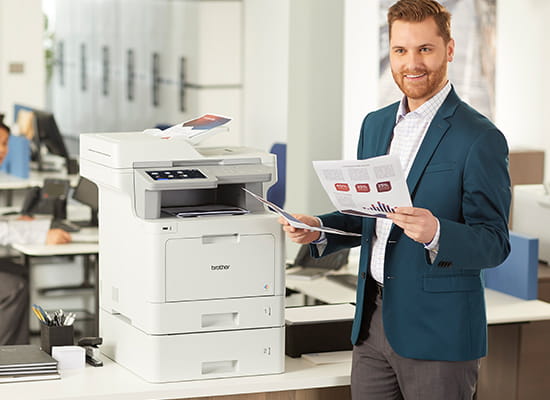This photograph captures a lively office scene with a man as the focal point, positioned toward the right side of the frame. The man, sporting a teal blue jacket and a checkered button-up shirt, has reddish brown hair, light-colored eyes, and a close-cut beard and mustache. He smiles enthusiastically while holding two pieces of paper. One paper, held in his left hand, displays a bar graph and colorful boxes, indicating it is likely a report with statistical data.

Adjacent to the man is a beige, multi-tiered Brother printer, which is actively printing out a colorful page. The printer, featuring stacked trays, dominates the corner of a cluttered desk. Office supplies such as a stapler, and a container of pens and pencils are scattered around the printer area.

In the softly blurred background, there is a woman sitting at her desk, observing the man. Her workspace includes a telephone and a computer, contributing to the bustling office atmosphere. Further back, a row of lockers or servers lines the wall, rounding out the busy office setting.